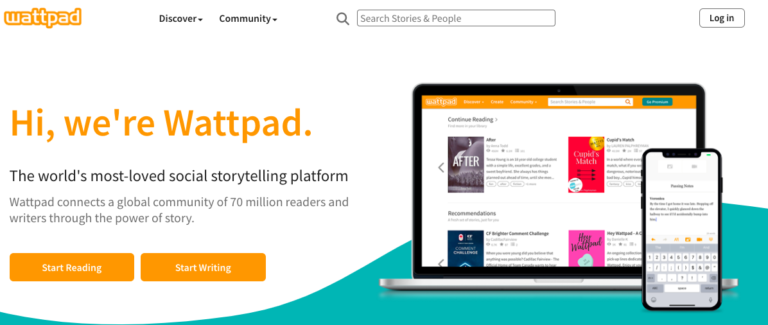The image captures a screenshot of the Wattpad website's homepage. Located in the upper left-hand corner, the Wattpad logo is displayed prominently in orange. Adjacent to the logo are navigation options including "Discover" and "Community," each accompanied by a drop-down menu. A search bar is placed centrally, while on the right-hand side, there is a login box.

Dominating the page is a large, bold orange header that reads, "Hi, we're Wattpad, the world's most loved social storytelling platform. Wattpad connects a global community of 70 million readers and writers through the power of story." Directly beneath this tagline are two orange buttons labeled "Start Reading" and "Start Writing," designed to attract user engagement.

To the right-hand side of this central messaging, an illustrative image showcases both an iPhone and a laptop displaying the Wattpad website. The laptop reveals four book covers in different colors—black and white ("After"), red, blue, and pink, though the titles of the latter three are too small to decipher. On the iPhone screen, the website interface is depicted, featuring only text and minimal graphics including smiley faces and the keyboard, emphasizing the platform's accessibility across devices.